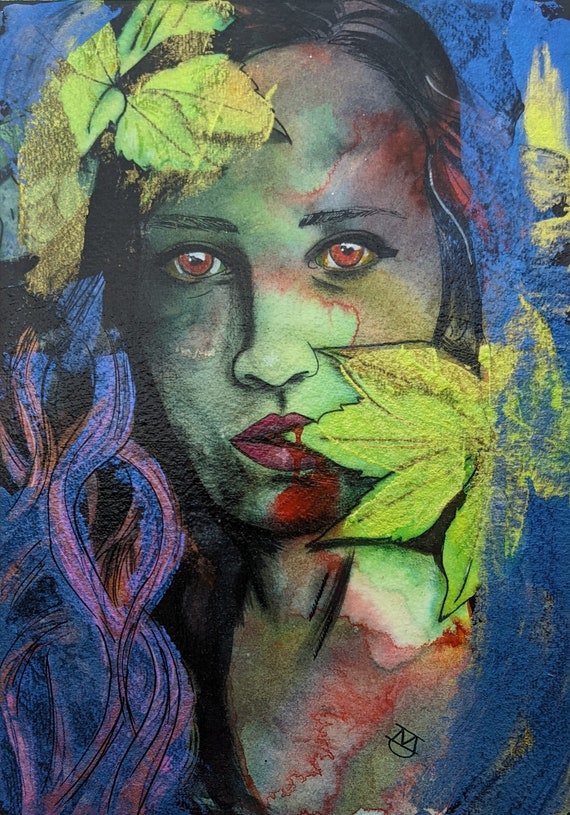This is a detailed, color acrylic painting of a young woman's face. She faces the viewer directly, with red eyes that create a striking gaze, and her lips are painted a vivid red. Her long, dark hair transitions into shades of blue and pink on the sides, and on the bottom left, it swirls into a stylized shape. Yellow leaves cover parts of her face, adding an abstract and intriguing element; one leaf is at the top left of her head and another near the bottom of her face. The background features a gradient of blue colors, complementing the bleeding of red and brown hues on her chest, chin, and forehead, which gives a dramatic, almost vampiric effect. The overall color palette is both vivid and surreal, emphasizing the contrast between the natural elements and the abstract use of colors. A subtle artist's signature, a stylized 'M', is located at the very bottom of the painting. The piece does not include any other figures or animals, focusing entirely on the woman's enigmatic and expressive face.